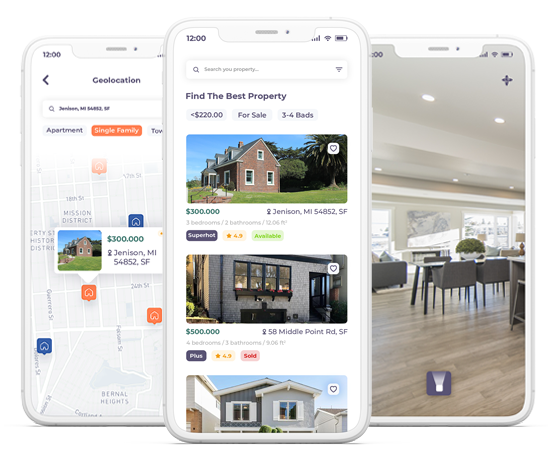The image displays three distinct cell phone screens, each outlined clearly. 

On the left screen, the top-left corner indicates the time as 12:00. Directly below that is a label stating "geolocation," followed by a search bar with an address entered. There are three category tabs underneath: the left tab is labeled "apartment," the middle tab has an orange background and is labeled "single family," while the right tab is obscured. Below these tabs is a light gray map featuring white roads and some street names. A highlighted location, marked with a picture of a house and a front yard, displays a price of $300,000.

The center screen shows the time at the top with a battery icon on the right. Below this is a search bar, followed by the phrase "find the best property." Three labels are shown below: the middle label indicates “$220 for sale,” and another reads “three to four beds.” Further down are three house listings; the top two listings display the price and address beneath corresponding images of houses.

The right screen features an interior view of a home, showcasing hardwood flooring, black furniture, and a greenhouse plant. The ceiling is gray, and windows are visible in the background. A purple box at the bottom of the screen contains a flashlight icon.